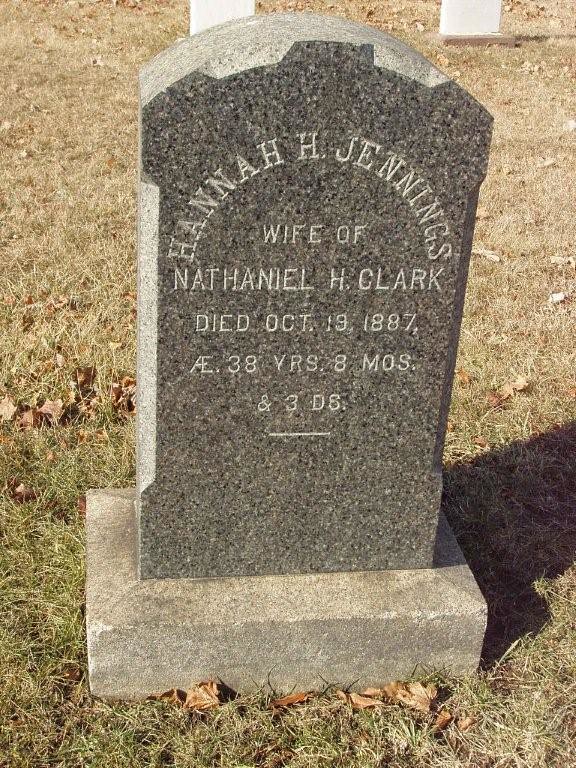The photograph, taken on a sunny winter day, captures a gray marble tombstone set on a concrete slab within a cemetery. The surrounding landscape is characterized by wilted, semi-dead grass with patches of brown and occasional fallen leaves, composing a somber scene. The tombstone prominently displays the name "Hannah H. Lennings" etched in a semi-circular arc at the top. Below, in horizontal lines, the inscription reads: "Wife of Nathaniel H. Clark, died October 19th, 1887, aged 38 years, 8 months, and 3 days." The tombstone itself features a rectangular base supporting a rectangular upper section capped with a gentle arch. To the left third of the image and a few inches in from the right, two other gravestones are visible, appearing white against the muted backdrop. The luminous winter sun accentuates the text and textures, adding depth to the melancholic atmosphere.